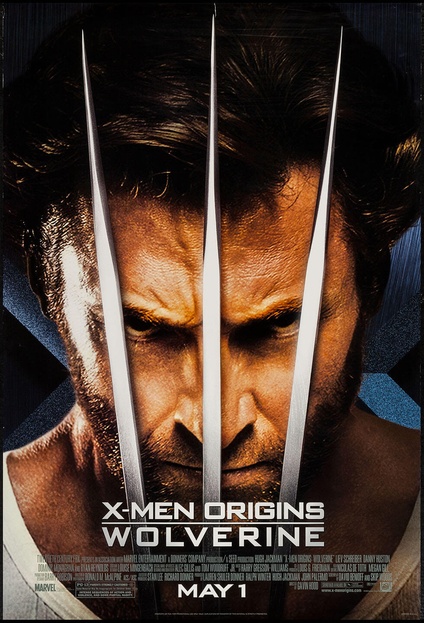This image is a highly detailed movie poster for "X-Men Origins: Wolverine," prominently featuring Hugh Jackman as Wolverine. The rectangular poster centers on a dramatic close-up of Wolverine's face, neck, and hand. His intense, golden-eyed gaze meets the viewer through the three metallic claws protruding from his fist, which cover his entire face. Wolverine's distinctive hairstyle, beard, and mustache are clearly visible. He is depicted wearing a white V-neck t-shirt, though the shirt and his shoulders are mostly obscured by the framing and the darkness of the background. The top of the poster blends seamlessly into a black backdrop with hints of blue. At the bottom, the poster displays the title "X-Men Origins: Wolverine" in bold white text, along with the release date "May 1st." Marvel's logo is present on one side, alongside the typical array of credits and information found on movie posters.